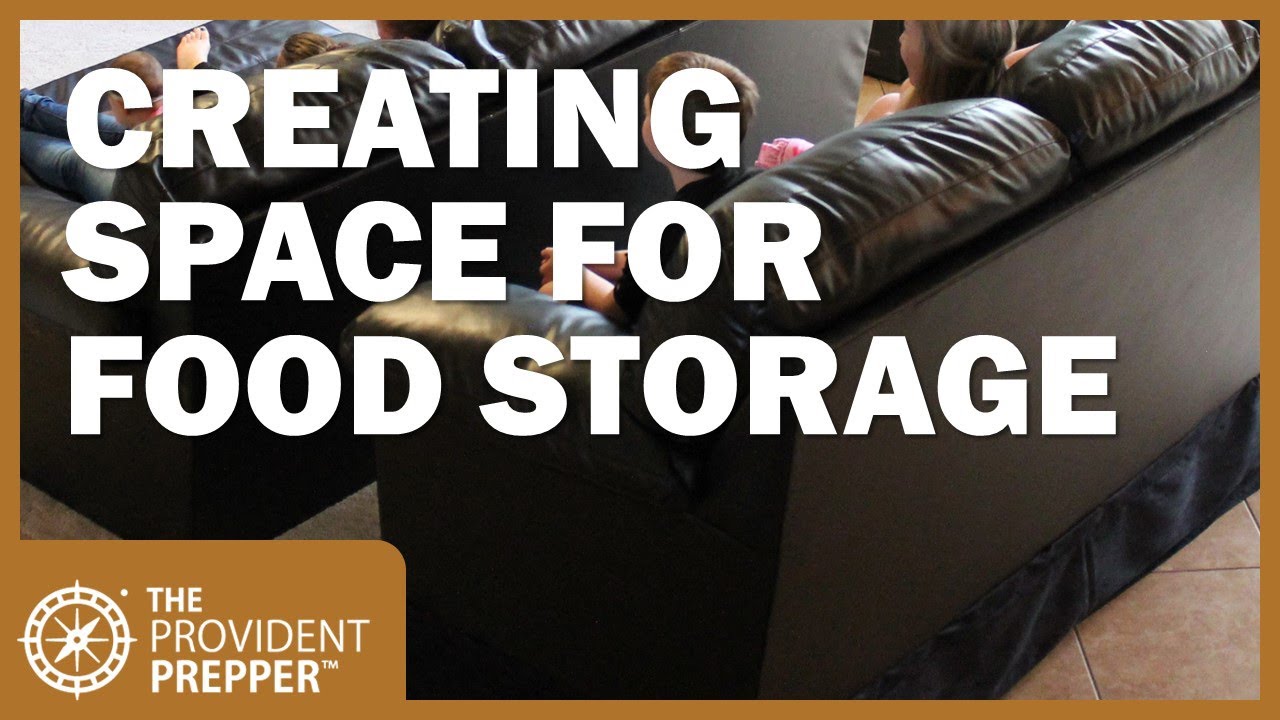The image features bold, white text that reads "Creating Space for Food Storage" prominently in the left-hand corner, dominating the top half of the image. This text overlays a scene depicting a family gathered on a black leather couch, which occupies the foreground and continues into a second row of similar furniture in the background. The family appears to include a child, a woman beside him, and several other individuals, with at least one of the children sitting barefoot. The room has a tiled floor and a brownish-orange background that curves into a rectangular shape. Additionally, the bottom left corner of the image displays a white compass emblem and the text "The Provident Wrapper" accompanied by a trademark logo, contributing to a sense of branding and context for the scene.